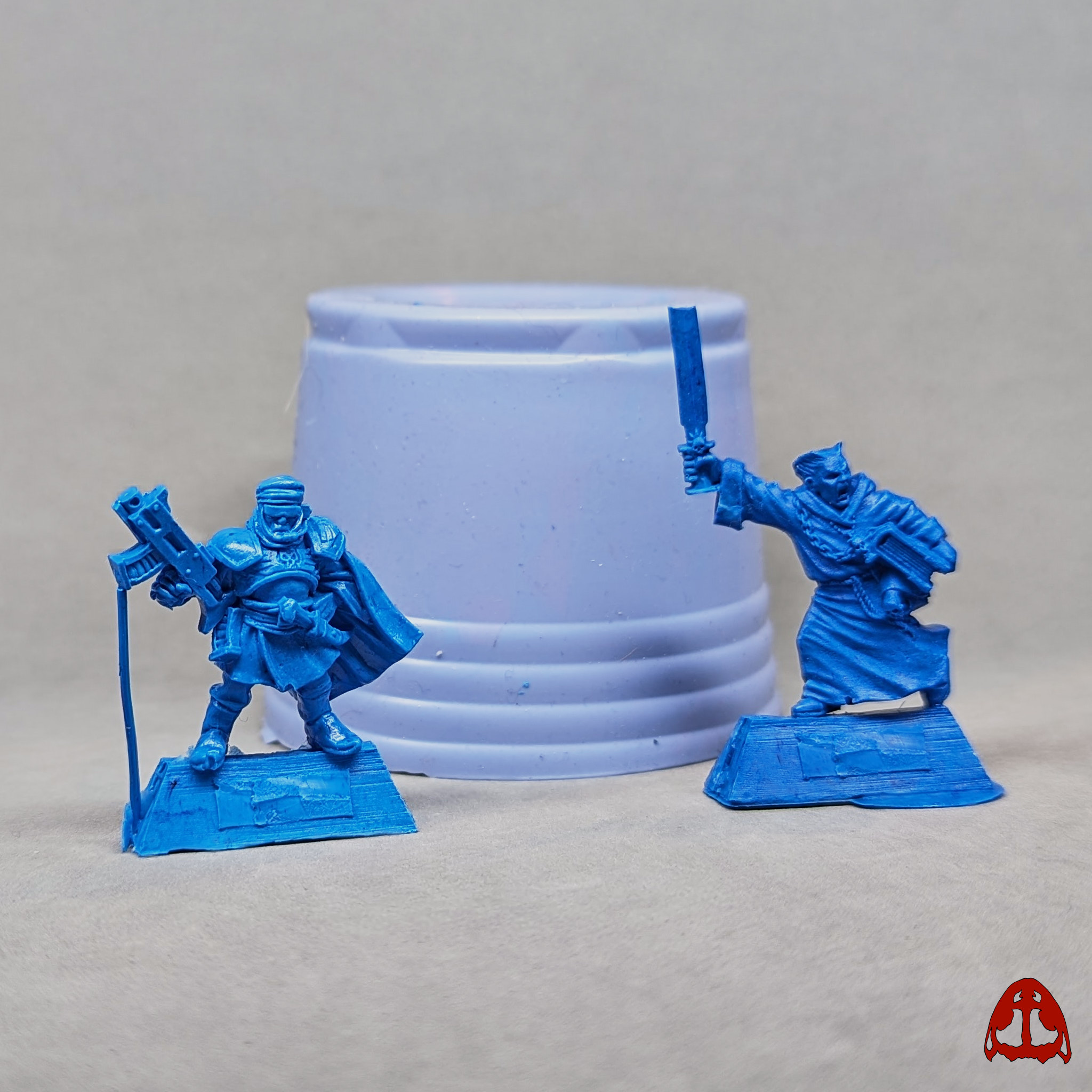This is a detailed photograph of two small, turquoise-blue figurines likely produced using a 3D printer, evident from the visible printing imperfections. Both figurines are positioned on individual, trapezoidal platforms and are facing the viewer. 

The figurine on the left is a warrior characterized by his robust build and ornate gear. He wears a helmet, thick goggles, and a large cape that flows behind him. His outfit includes combat boots and protective armor on his shoulders. He stands with legs apart, clutching a large machine gun in his right hand, which is supported by a prop to maintain its position. A dagger is strapped to his belt, and he appears ready for combat.

The figurine on the right represents a commanding figure, dressed in long, flowing robes reminiscent of a Roman toga, complete with scrolls and a tome held beneath his left arm. His long robe reaches the ground, and his hair is styled in an angular, flat-top fashion. With an intense expression and mouth open as if yelling, he raises a broad, square-edged sword vertically with his right hand. 

Both figures are staged in front of a seamless, gray lightbox backdrop, adding a professional display feel. Behind them sits an overturned blue cup or small pot, providing a sense of scale. At the bottom right of the image is a red logo that appears emblematic but lacks readable text.